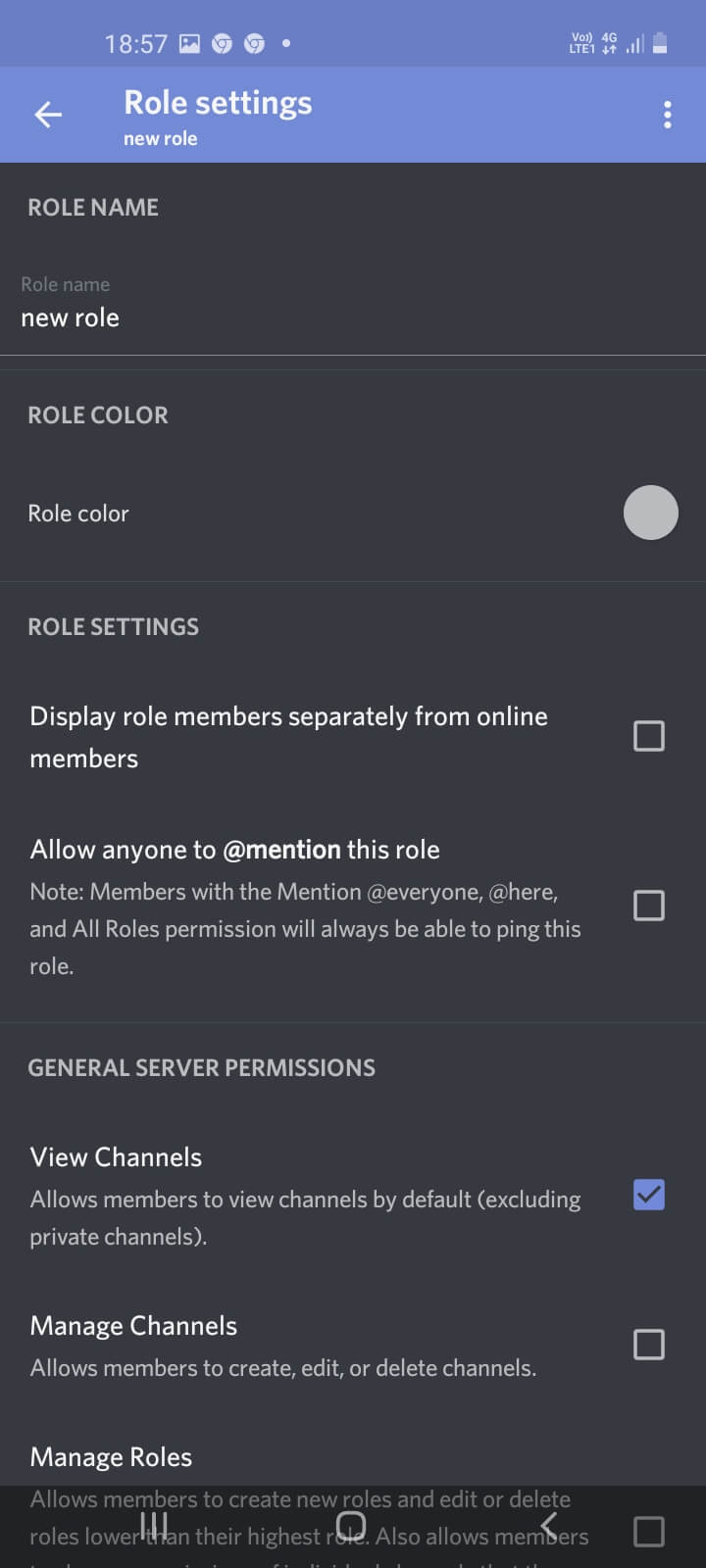This image is a detailed screenshot from a cell phone, as indicated by the presence of a battery icon, a series of small icons, and a timestamp at the top of the screen. Directly below this top bar, there is a light blue bar with white text displaying the words "Role Settings" and "New Role," alongside an expand and contract button.

The main content of the screenshot showcases a user interface for managing permissions related to a website. This interface allows users to perform a variety of tasks including adding new roles, modifying existing roles, and changing the colors associated with different roles to highlight certain functionalities. Furthermore, users can display role members to keep track of who has access to various parts of the website. The interface also includes features to check for any external mentions of the site, ensuring comprehensive role management and security. This role settings menu is a generic tool used across various websites for handling permission-related tasks efficiently.